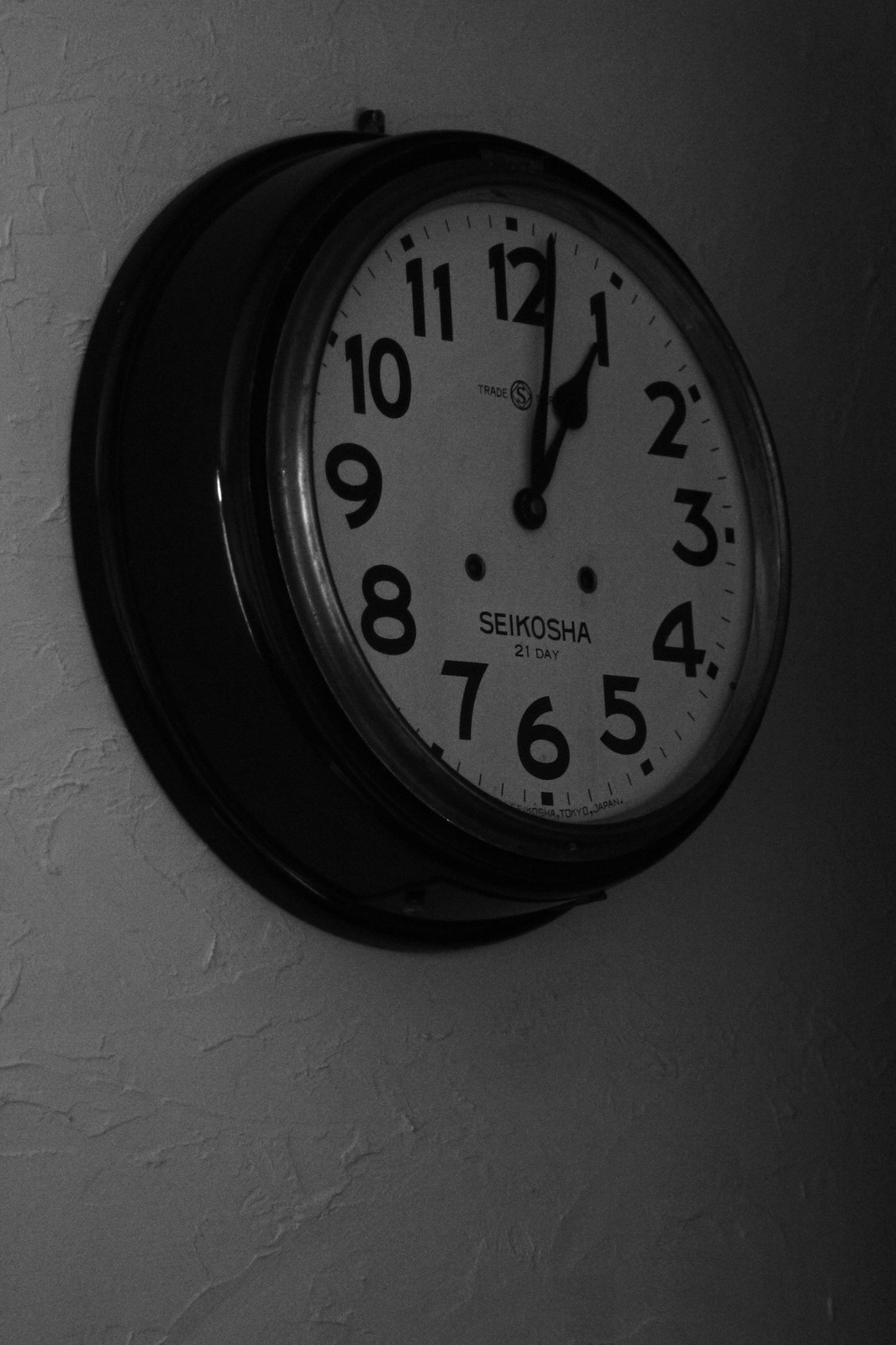This black and white photograph depicts a classic wall clock mounted on a textured plaster wall, likely a knockdown texture. The clock features a thick, shiny black frame and a glass-covered face. The face of the clock is an off-white color and displays bold black numbers, ranging from 1 to 12, with additional small markings for precise time indication. The clock's hands are black, including a long minute hand pointed at the 2 and a short hour hand at the 1, indicating the time as 1:02. Notably, the clock lacks a second hand. Towards the bottom-center of the clock face, the words "Seiko Sha" and "21 day" are printed in black. The overall lighting of the photograph is dark, with only a minimal amount of light coming from the left side, contributing little illumination to the scene.